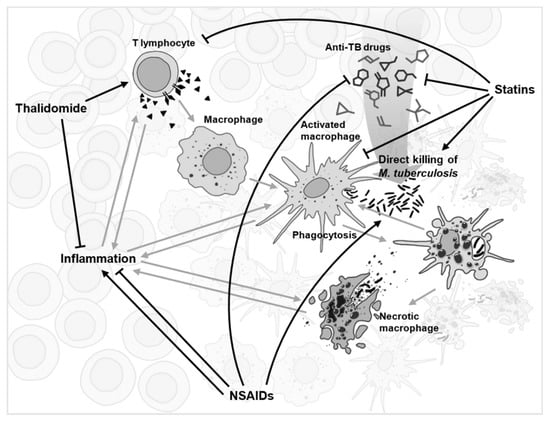This detailed diagram, presented in a rectangular, landscape format, is rendered in black and white with gray tones. At the bottom center, the term "NSAIDs" is prominently displayed, with arrows extending horizontally to both the left and right.

On the left side of the diagram:
- Directly above the leftward arrow, the term "inflammation" is written.
- Positioned above "inflammation," the word "thalidomide" is shown.

On the right side of the diagram:
- Immediately to the right of the rightward arrow, "T lymphocyte" is noted.
- Below "T lymphocyte," the term "macrophage" appears.
- Adjacent to "macrophage," there is an indication of "activated macrophage."
- Above the "activated macrophage," the phrase "anti-TB drugs" is placed.
- Extending further to the right, the term "statins" is labeled, accompanied by four arrows diverging in different directions.
- Below "statins" and slightly to the left, "direct killing of M. tuberculosis" is specified.
- In the lower left corner, we find "phagocytosis."
- To the bottom right of "phagocytosis," the term "necrotic macrophage" is documented.

Throughout the diagram, symbols are situated adjacent to several of these terms, presumably representing various biological processes or interactions.